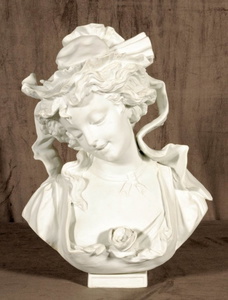This detailed photograph features a finely crafted white marble bust of a female figure, prominently displayed against a coffee-colored wood backdrop. The bust is set on a rectangular white base. It depicts an intricately carved woman adorned in a low-cut dress that wraps over her angled shoulders. At the center of the dress's fold on her chest, there is a detailed carving of a rose. Around her neck, a white ribbon is delicately tied, giving a sense of elegance. The figure's head is slightly tilted downward and to the left, with closed eyes and a gentle smile, exuding a serene and content expression. Her hair flows gracefully on both sides, pinned up and topped with a pleated white hat that has intricate strips of cloth cascading in an 'S' shape along her shoulders. The intricate craftsmanship highlights not only the facial features but also the elaborate clothing and accessories, making it an exquisite and lifelike representation.